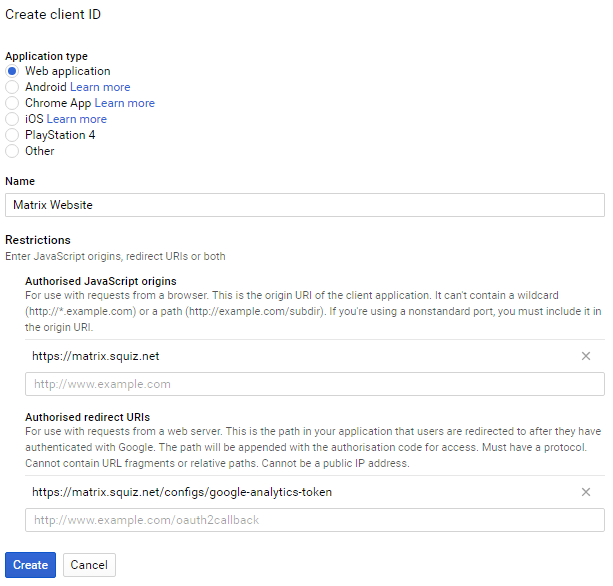Illustrated in the image is a user interface for creating a client ID for an application. The header reads "Create Client ID," followed by a section labeled "Application Type," with "Web Application" selected by default. Under this, there are options to learn more about different application types such as "Android," "Chrome App," "iOS," "PlayStation 4," and "Other."

Further down, there is a field labeled "Name" with a long rectangular input box containing the placeholder text "Matrix Website." Below this, a section titled "Restrictions" provides fields for entering authorized JavaScript origins and redirect URIs or both. Detailed instructions indicate that the authorized JavaScript origins support requests from a browser, specifying the format and constraints, such as not containing a wildcard and the inclusion of the port if it's nonstandard. An example URL given is "https://matrix.squiz.net" followed by "http://www.example.com."

Additionally, the section provides guidelines for authorized redirect URIs for web server requests, detailing that it must have a protocol, cannot include URL fragments or relative paths, and cannot be a public IP address. An example provided is "https://matrix.squiz.net."

At the bottom of the interface, there are two buttons labeled "Create" and "Cancel," giving users the option to either proceed with creating the client ID or cancel the operation.